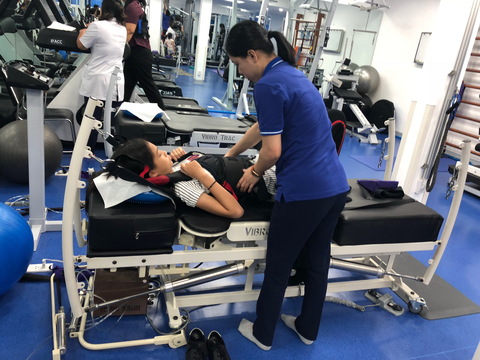In a brightly lit physical therapy room with smooth blue reflective flooring and white walls lined with various exercise equipment, a detailed scene unfolds. At the heart of the photograph, a woman in white socks, black pants, and a blue polo with white striped accents on the collar and sleeves is focused on assisting another woman lying on a black padded weightlifting table. This table, which is covered with black mats and equipped with various chains and straps, appears to be part of a rehabilitation setting. The woman lying down is wearing a vest with straps connected to a metal frame attached to the table. Both women, who appear to be of Asian descent, are engaged in what seems to be a physical therapy session, with the standing woman adjusting the other's vest with both hands placed on her chest. Nearby, there are yoga balls and additional exercise equipment. In the background, a nurse or physician with shoulder-length black hair, dressed in a white short-sleeve jacket, oversees the room. Additionally, an individual wearing a dark red shirt and black pants is seen using a treadmill, adding to the bustling yet focused environment of this rehabilitation facility.